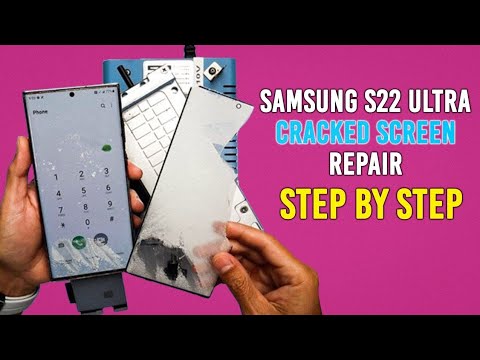The thumbnail for a YouTube video or website features a vividly detailed composition against a pink background, with black horizontal borders at the top and bottom. Centrally, a pair of black hands prominently holds a damaged Samsung S22 Ultra phone. The left hand grips the phone, which displays a dialing pad with numbers 1 through 0 and additional keys. The right hand holds what appears to be a shattered screen protector or glass cover detached from the phone. Accompanying the image are texts: "Samsung S22 Ultra" in white, "Cracked Screen" in blue, "Repair" in white, and "Step by Step" in yellow, all on the right side of the image. Notable elements beneath the hands include what might be repair equipment, adding context to the step-by-step repair theme. The background contains a hint of a light blue tablet and a white scheduling calendar, subtly included between the depicted phone and the broken screen.